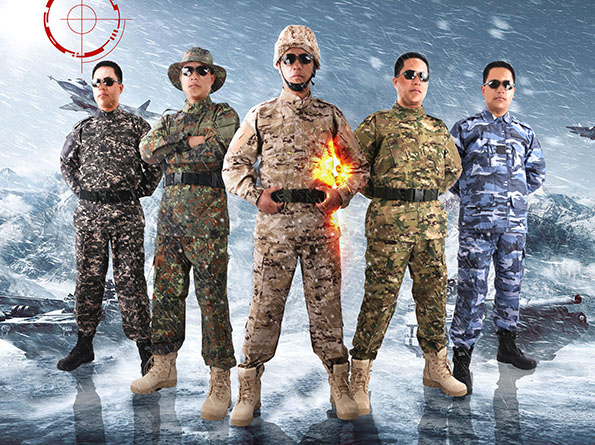The image features five individuals prominently positioned in the center, dressed in various military uniforms representing different branches of the military. They stand on a reflective blue and white ice-like surface, set against a backdrop of computer-generated snowy mountains, with drifting snow adding to the wintry environment. In the upper left corner, there is a target-like logo. The men wear hats and sunglasses, adding to the uniformity despite their differing attires. Each uniform varies, with the central figure donning a tan and brown camouflage, flanked by others in green classic camo and arctic blue camo on one side, and dark olive green and brown camouflage with black and tan digital camo on the other. The scene includes additional military elements such as a tank and airplanes in the background, suggesting a promotional or recruitment purpose for military service. The colors present in the image include red, white, blue, brown, green, silver, gray, and black, emphasizing the range and diversity of military attire and gear.